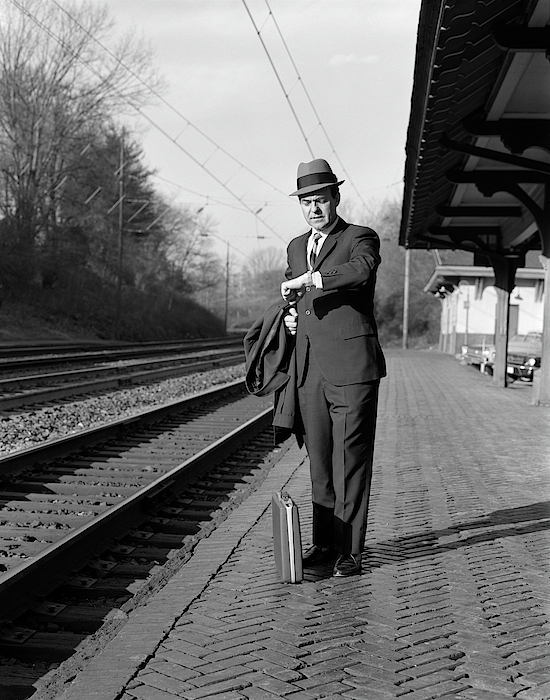This black-and-white photograph depicts a well-dressed gentleman from perhaps the 1950s, standing on a brick platform at an outdoor train station during the daytime. He is positioned in front of a train depot, partially visible with its metallic and wooden awning providing shelter. In his left hand, he checks his wristwatch with a somewhat concerned expression, possibly due to the train's delay. He wears a suit, a tie, a buttoned jacket, and a hat adorned with a black band, adding a touch of business formality to his appearance. His overcoat is draped over his right arm. Directly at his feet lies a thin, rectangular briefcase with silver trim. The platform, flanked by three empty railroad tracks and scattered with stones, also features overhead electrical lines and utility poles. In the distance, dormant trees stretch their bare branches against the sky. To the right, parked cars and a building with a color base transitioning to white at the top form the backdrop of this solitary scene, enhanced by the man's pronounced shadow on the brick surface.